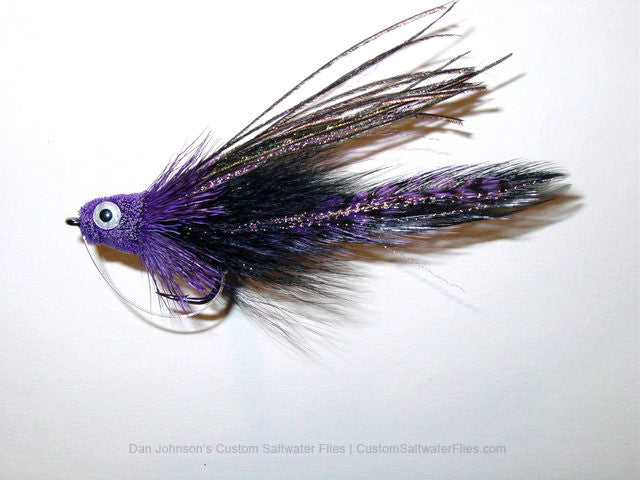This photograph showcases a meticulously crafted fishing lure, known technically as a "saltwater fly," set against a gradient white-to-gray background. At the center left of the image is the saltwater fly, characterized by its uniquely designed features. The head of the lure is purple, textured, and adorned with a silver, googly eye that has a black center. Emanating from the head are various materials including threads, furs, and multiple feathers in shades of purple, brown, and black. A notable feature is a prominent, long purple feather that extends from the center, flanked by thinner, darker feathers. Extending from the bottom of the head, a black hook is visible, curling towards the left. Additionally, a black ring attached to the head signifies the point where a fishing line can be connected, with part of the line curling beneath the lure. Below the lure, the text reads: "Dan Johnson's Custom Saltwater Flies, CustomSaltwaterFlies.com," confirming the lure’s purpose and craftsmanship origin. This detailed construct not only emphasizes the artistic intricacies of the lure but also highlights its functional aspects as a specialized fishing tool.